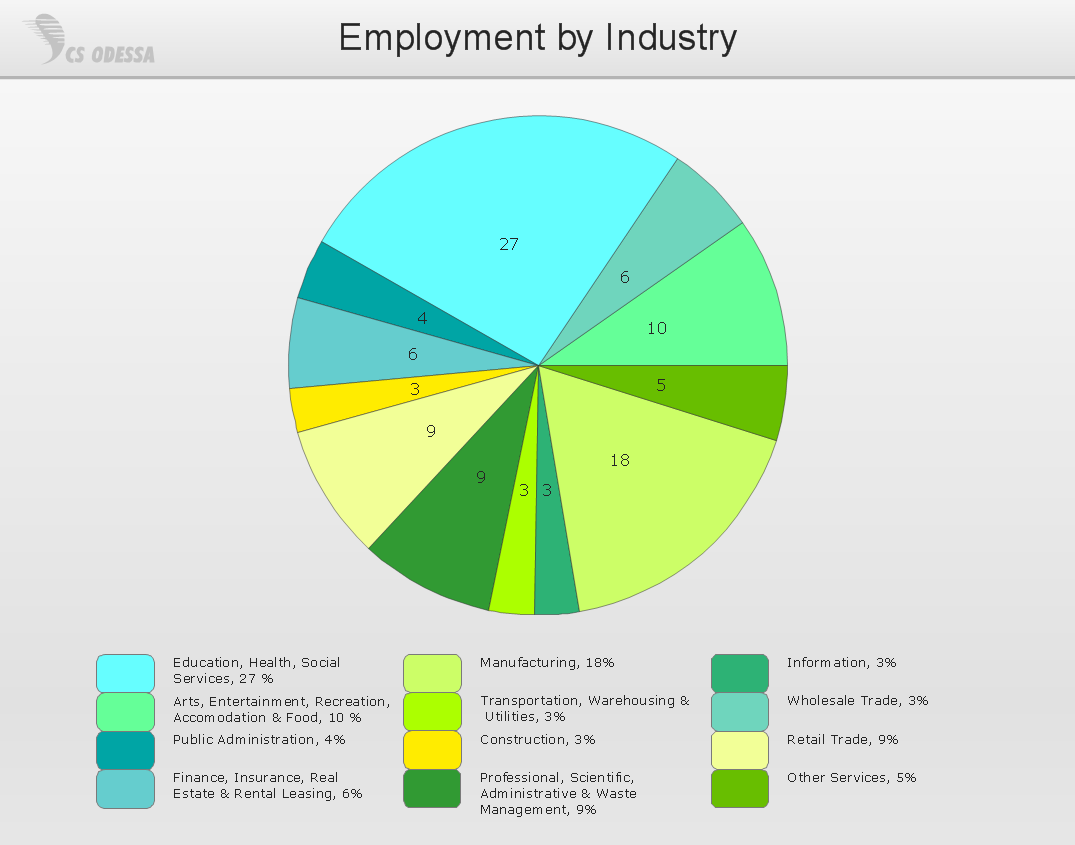The image depicts a pie chart titled "Employment by Industry," centered at the top in black text against a light gray background. On the top left, there is a logo that reads "CS Odessa," slightly darker than the background. Below it, a horizontal rule separates the heading from the chart. The pie chart itself features various colors, primarily cool tones with shades of green, turquoise, and yellow, each representing different industries. The chart details the following employment sectors: Education, Health, and Social Services at 27% in light turquoise; Arts, Entertainment, Recreation, Accommodation, and Food at 10% in light green; Public Administration at 4% in teal; Finance, Insurance, Real Estate, and Rental Leasing at 6% in darker turquoise; Manufacturing at 18% in light lime green; Transportation, Warehousing, and Utilities at 3% in darker lime green; Construction at 3% in bright yellow; Professional, Scientific, Administrative, and Waste Management at 9% in deep green; Information at 3% in emerald green; Wholesale Trade at 3% in medium turquoise; Retail Trade at 9% in light yellow; and Other Services at 5% in medium greenish-yellow. The percentages are marked on each slice corresponding to a color-coded legend at the bottom of the chart.